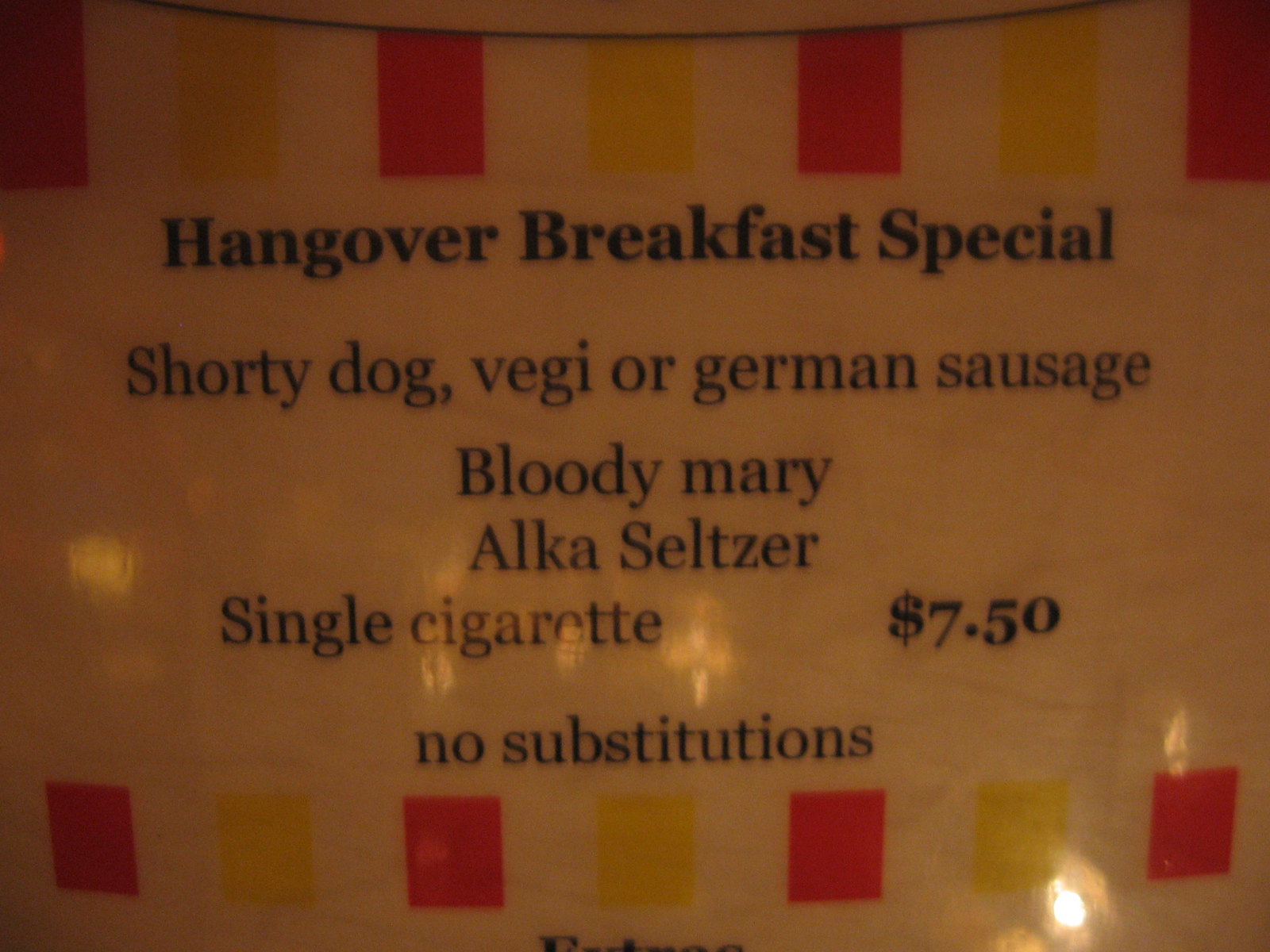This dimly lit image appears to be an advertisement or menu placed in a bar or restaurant, evidenced by the reflections indicating the use of flash. The background is a yellowed, laminated piece of paper adorned with a decorative design: red and yellow flags strung across the top, and red and yellow squares lining the bottom, though the yellow squares are less discernible due to the lighting conditions. The central text, framed by these decorations, prominently features the offer: "Hangover Breakfast Special." Below this headline, the details read: "Shorty Dog Veggie or German Sausage, Bloody Mary, Alka-Seltzer, and a single cigarette for $7.50. No substitutions." The laminate material of the page catches the reflections of ambient lights, adding to the somewhat nostalgic appeal. The overall scene suggests a cozy, perhaps vintage setting typical of a dimly lit bar or intimate dining venue.